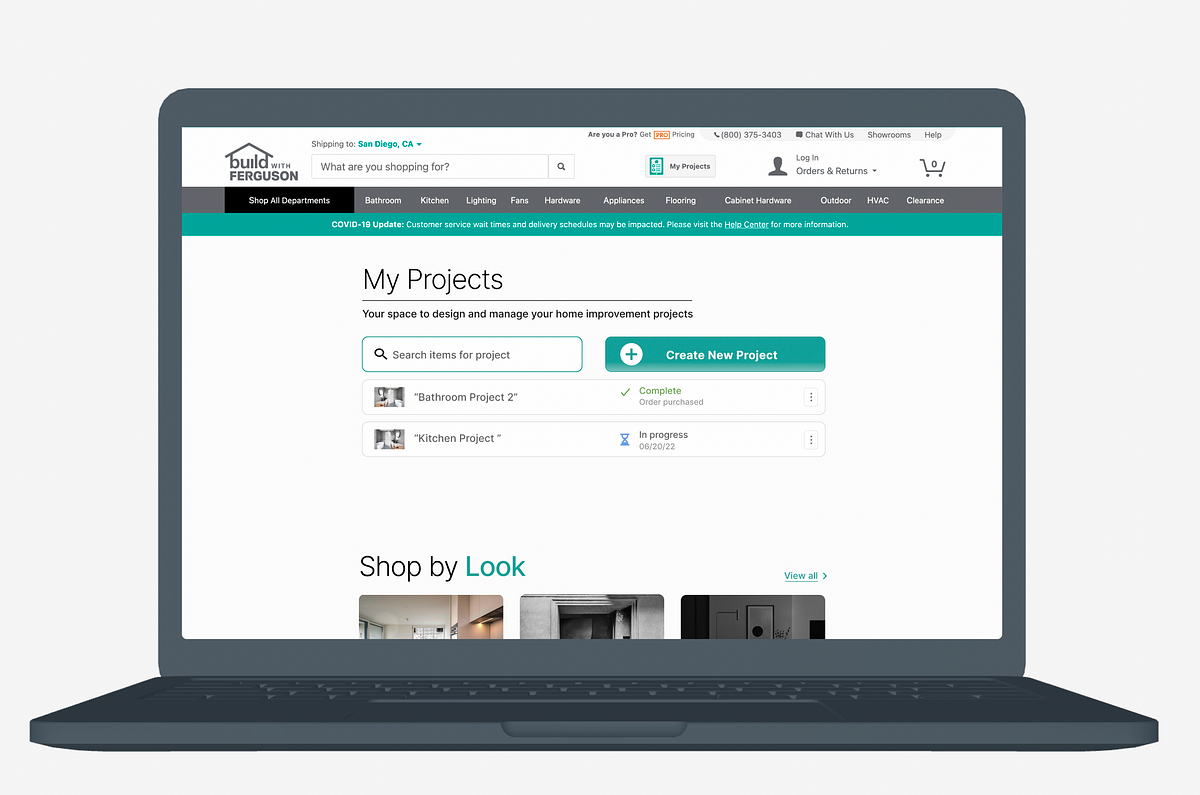This image features a sleek black laptop, reminiscent of a MacBook, prominently displayed against a pristine white background, making it ideal for a sales page. The screen showcases a web page from "Build with Ferguson." At the top of the interface is a dark grey navigation menu, complemented by a green ticker tape directly underneath. The main area of the page features a clean white background with black text and green buttons for optimal readability. At the top of this section, there is a "My Projects" header, accompanied by a text field and a "Create New Project" button. Beneath this, a "Shop by Look" section is evident, though the page design partially obscures three photographs at the bottom. This meticulous setup aims to blend the elegance of the device with the functionality of the website.